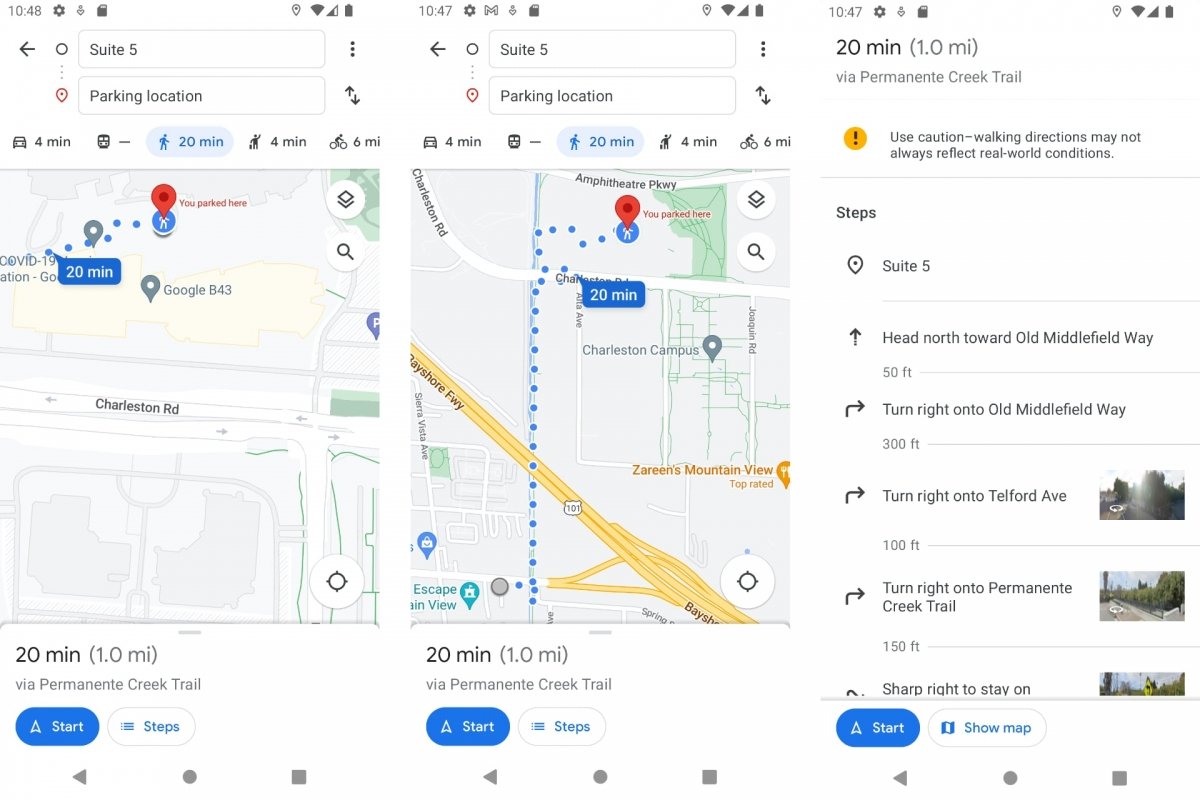A set of three side-by-side images displayed on a cell phone screen, capturing a search result for walking directions. The timestamps on the images are 10:48 and 10:47 AM. The first two images show a map with the chosen walking route and the estimated time to reach the destination, indicating that it will take 20 minutes to walk one mile. The third image provides a detailed, text-based step-by-step guide for the walking route, starting from "Suite 5" and listing subsequent directions.